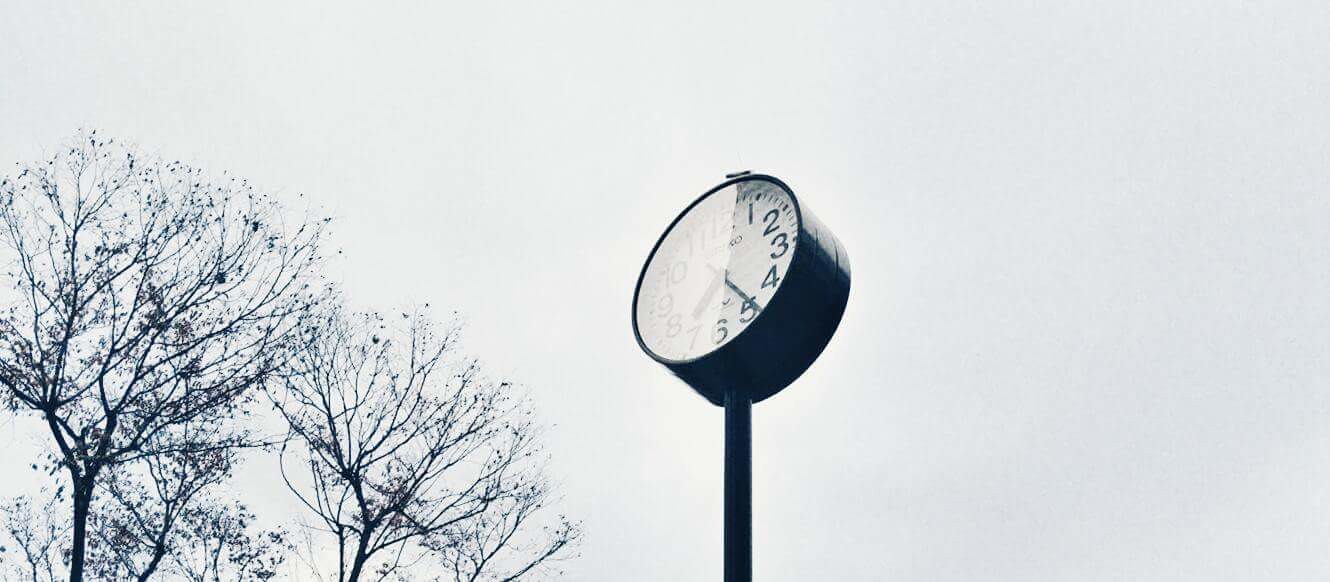This black-and-white photograph captures an upward view of a round clock perched atop a black pole. The clock, positioned centrally in the image, features a white face with black standard numbers and minute marks. Both the hour and minute hands indicate a time of approximately 7:25. The left half of the clock face is partially obscured by a reflection or light distortion, making the numbers less visible. Surrounding the clock, the sky presents a uniform gray, suggesting an overcast day. To the left, the tops of trees with sparse vegetation hint at an autumn setting, their bare branches reaching into the frame.